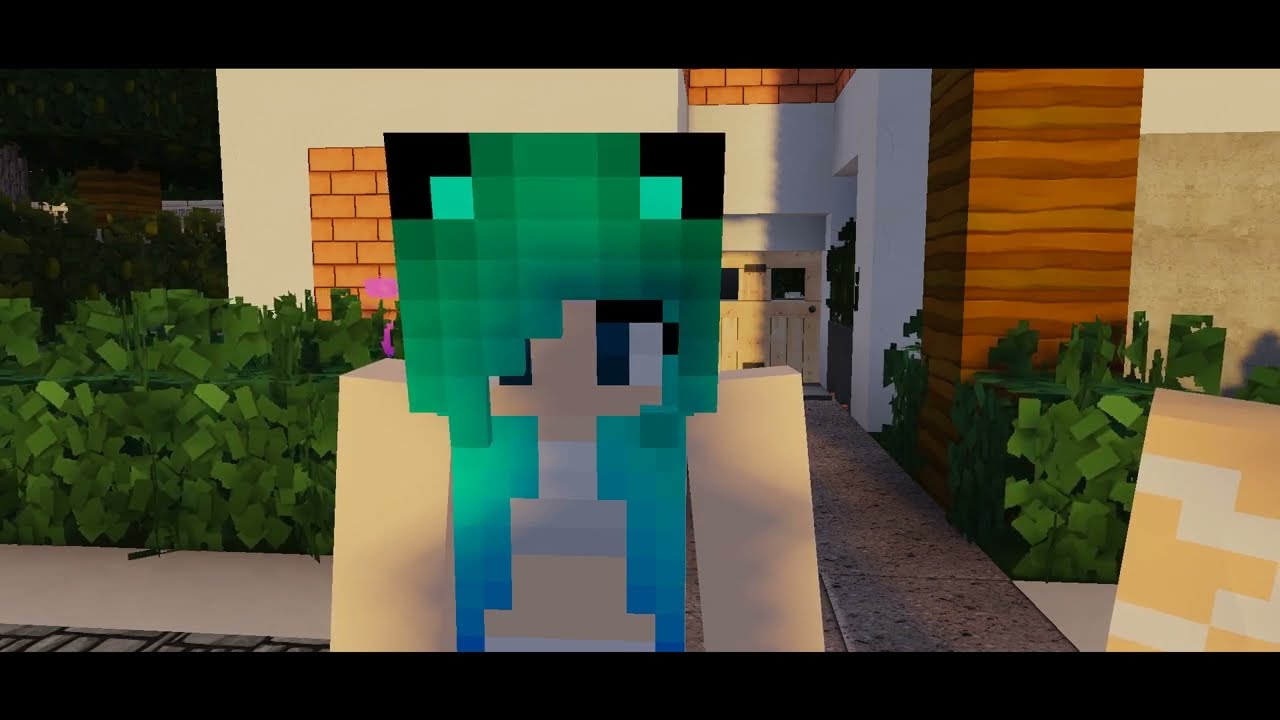In the image, we observe a digitally rendered scene resembling a video game, possibly Minecraft or a similar child-oriented game. At the center, there’s a large, multistory building with a mix of light and dark brown hues, suggestive of a hotel or residential complex. At the top-left of this building stands a character that appears to be from a Lego-like design. On the building’s left side, we notice a tall tree and faint clouds in a medium-blue sky, hinting at a peaceful setting despite the chaos. Emanating from the building's roof are elements that suggest a recent explosion, with visible smoke and flames.

The image is framed by black banners at the top and bottom. The text "Perfect Paradise" is prominently displayed towards the middle right, progressing from light blue to turquoise with an array of sparkles and stars around it. The color palette includes black, blue, green, tan, and brown, combining to create a dynamic and engaging visual scene.